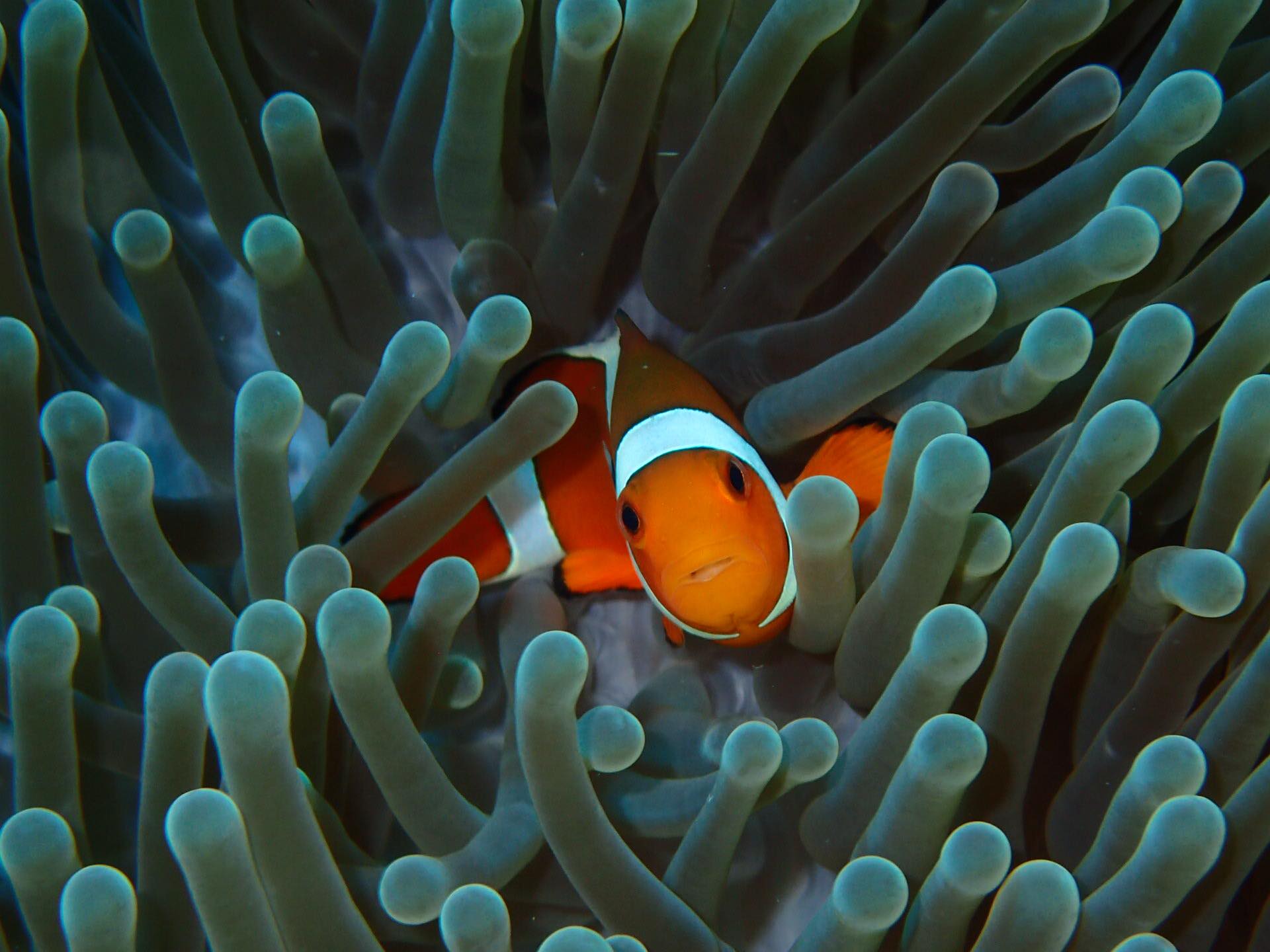The image displays an underwater scene reminiscent of a moment from "Finding Nemo." At the center of the square, full-color photograph is a bright orange clownfish, characterized by its distinctive white stripes edged with black. The fish, likely inspired by Nemo from the popular movie, has a noticeable worried expression as it looks upward. Surrounding the fish are various shades of green sea plants, which appear to be tube-shaped with lighter green bulbs at their tips, giving them a somewhat iridescent quality. The plants, possibly animated to resemble an undersea landscape, float and sway as if dancing in the water, contributing to the vibrant blend of green, orange, black, white, gray, and dark blue tones that dominate the scene. Taken outdoors with artificial lighting, this professional nature shot effectively captures the dynamic and colorful essence of an underwater world.